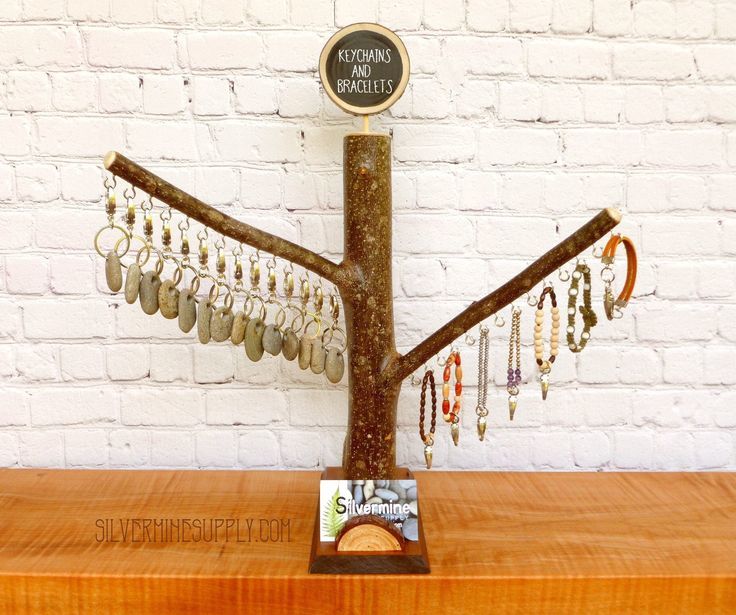The photograph captures a detailed display inside what appears to be a boutique shop, with a focus on jewelry and keychains. Central to the image is a small section of a tree trunk mounted on a thick wooden countertop, positioned against a white brick wall that has been painted over. The trunk features two branches, each serving as a display for different items. The left branch holds keychains made from natural, polished river stones, each stone oval-shaped and connected via metal rings to small golden hooks. The right branch showcases an array of colorful beaded bracelets, each made from a variety of vibrant stones. An informative circular sign at the top of the display reads "Keychains and Bracelets" with a gray background and a cream-colored border. At the base of the tree trunk, "silverminesupply.com" is prominently printed, indicating the store's name, Silvermine Supply. Additionally, a business card featuring the same name and website is placed at the front and center of the display, reinforcing the brand's identity. The overall scene exudes a rustic yet organized aesthetic, emphasizing the artisanal nature of the products.